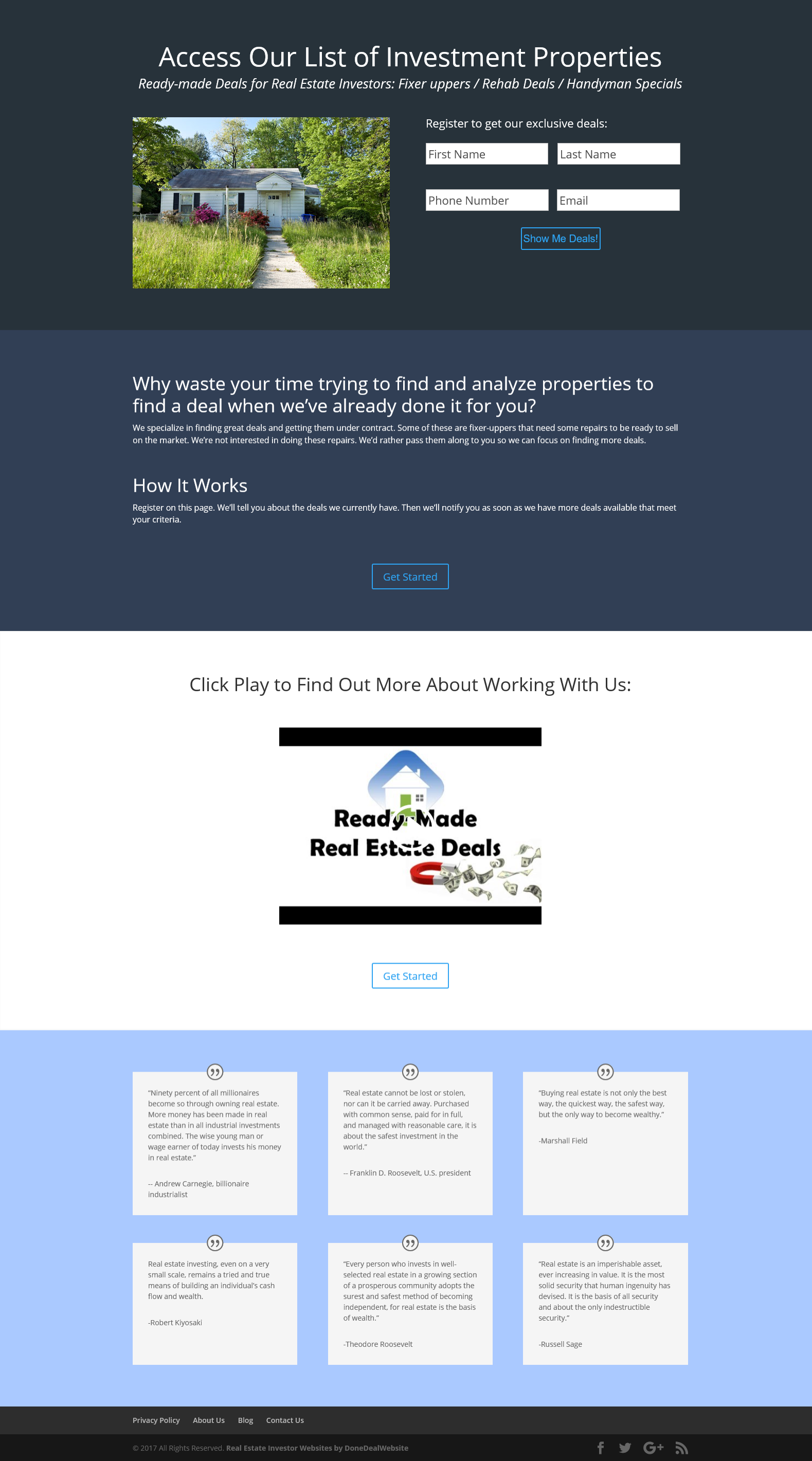The image features a promotional flyer inviting individuals to access a curated list of investment properties. The background of the flyer transitions from a dark blue at the top to a slightly lighter blue at the bottom. The main headline, "Access Our List of Investment Properties," is displayed prominently in white text.

The central part of the flyer emphasizes various types of investment opportunities, including "ready-made deals for real estate investors," "fixer uppers," "rehab deals," and "handyman specials." A picture of a house with overgrown grass further illustrates the type of properties available, suggesting that these are fixer-uppers requiring some work.

Below this, a registration form is presented, asking for the viewer's first name, last name, phone number, and email, with a call-to-action button labeled "Show Me Your Deals." An additional message encourages prospective investors not to waste time searching for and analyzing properties, as the deals have already been vetted.

The flyer also includes a "How It Works" section, although the details are too small to read. Another call-to-action button titled "Get Started" appears beneath this section. Towards the bottom, there's a video link with a play button for users to learn more about working with the company. Accompanying text, which is unfortunately too small to read, likely provides additional information and instructions.

The bottom section features testimonials, presumably from satisfied customers, although the text of these testimonials is also too small to decipher.